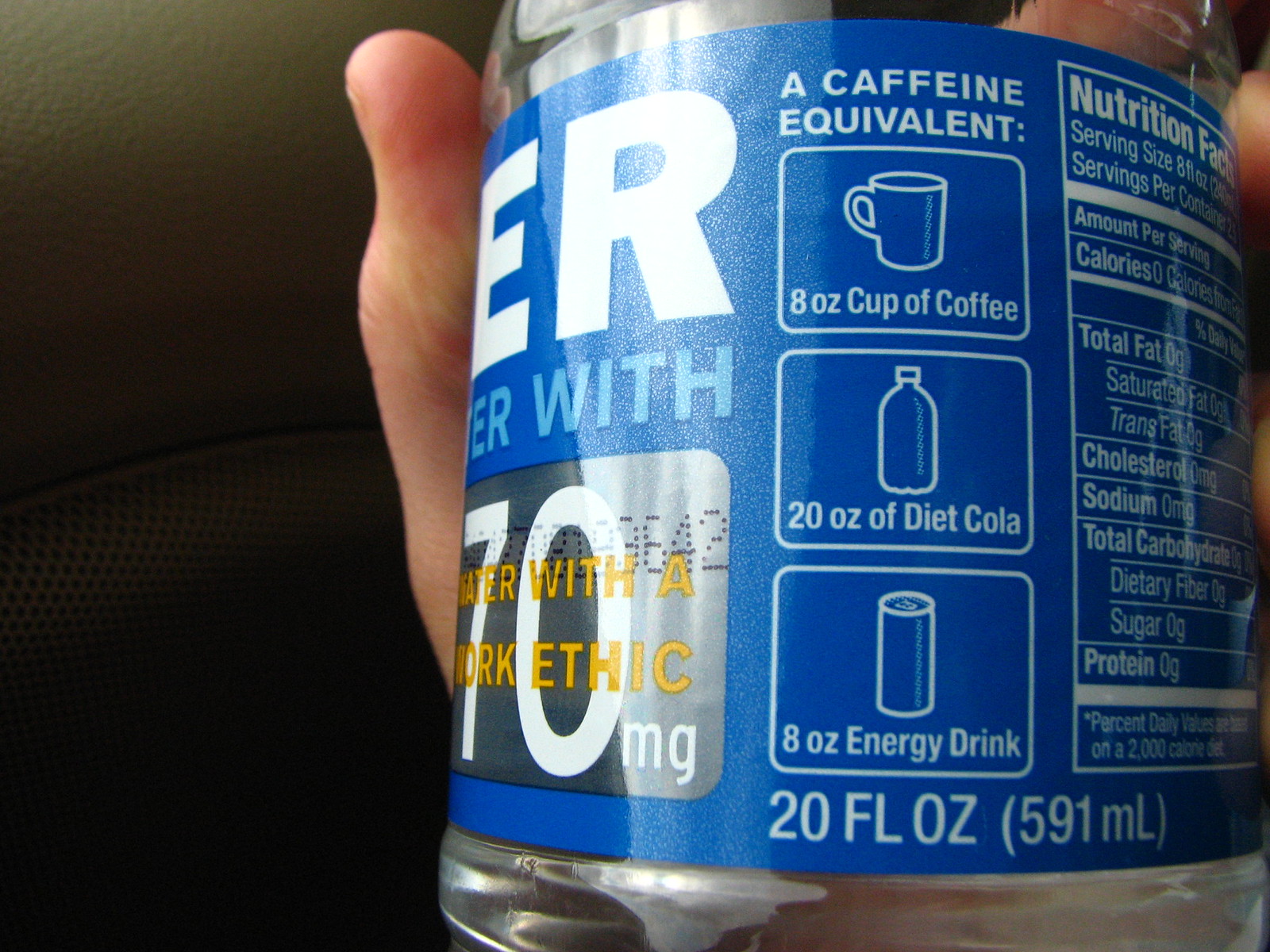The image is a close-up of a clear plastic bottle containing a beverage, potentially an energy or hydration drink. The focal point of the image is the blue label on the bottle, which prominently features a caffeine comparison. The label states "caffeine equivalent" and includes three small rectangular icons beneath it showing the caffeine content comparisons: an 8-ounce cup of coffee, a 20-ounce diet cola, and an 8-ounce energy drink. The bottle's size is indicated as 20 fluid ounces. The right side of the label shows partial nutrition facts with typical entries such as calories, cholesterol, sodium, total carbohydrates, and protein. The left side of the label displays large white letters "ER," which might be part of the word "water." The background of the image is dark, possibly black, with some gray tones suggesting it might be inside a vehicle. The person holding the bottle has their thumb visible on the left, and parts of three fingers can be seen on the right, with the bottle obscuring most of their hand. On the lower part of the label, there are additional details including "70 milligrams" in white and yellow lettering.